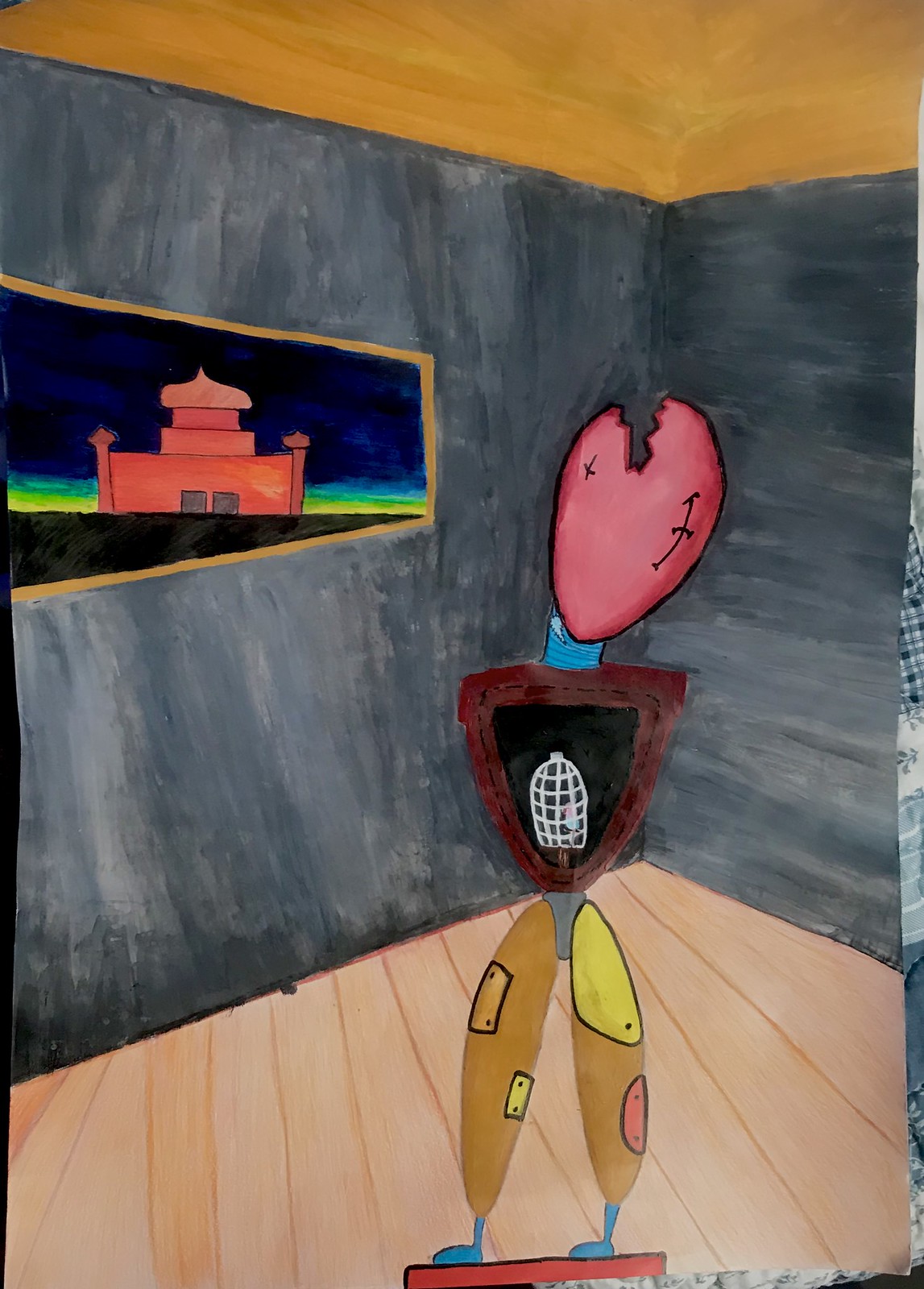Descriptive Caption: 

This hand-drawn artwork, possibly created by a student, features a unique and whimsical character. The person's head is shaped like a heart but with a jagged top and an X marked on it. Below the X, there's a vertical line intersected by another horizontal line. The character's neck is depicted as a blue spiral, adding an abstract touch. The body is a maroon upside-down triangle within which a birdcage-like pattern is drawn, evoking a sense of being trapped or constrained. The character is notably armless, enhancing its surreal appearance.

The lower body is intriguingly depicted; the legs resemble French bread baguettes in both color and shape, adorned with patches of yellow, pink, and tan. The feet are colored blue and drawn to face the same direction, contributing to the quirky aesthetic. This character stands on a wooden floor, set against a plain gray background. In the backdrop, there's a vibrant picture of a castle, colored pink, with a blue and yellow sky, adding a splash of color and fantasy to the scene.